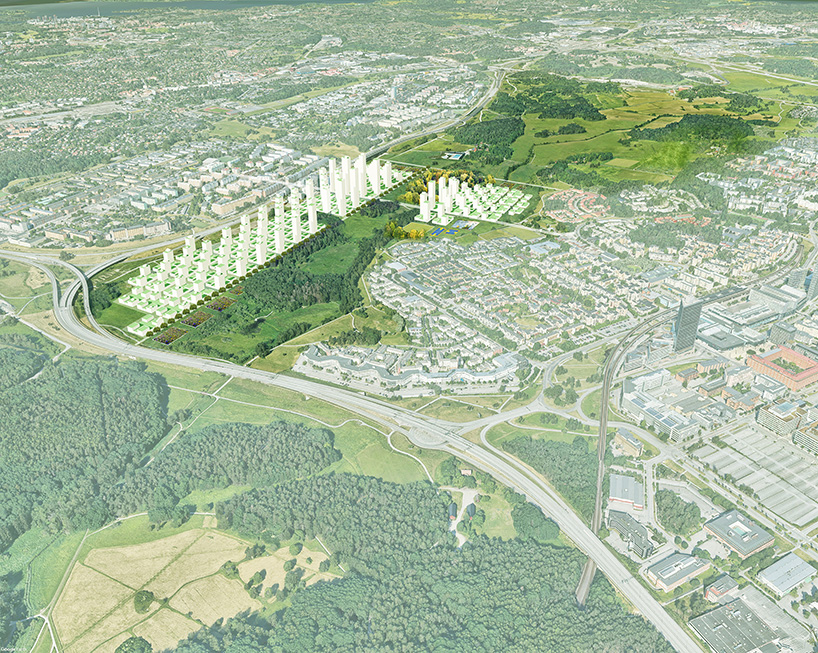This image is an aerial, possibly computer-generated, satellite photograph resembling a view from Google Earth. The cityscape below is a detailed mix of green, forested areas, urban city blocks, residential housing, and various buildings. The lower left portion features extensive forest patches interspersed with open fields. A distinct road curves from the lower right to the middle, extending toward the middle left, marked by a light gray color devoid of visible vehicles. 

The central and upper left sections of the image show a highlighted plot of land rich in green color, adorned with a dense patch of trees. Overlaying the photograph is a proposed development plan characterized by white, tall, thin buildings of varying heights, ranging from single-level to high-rise structures. These buildings form an L-shaped configuration, prominently displayed in the middle section and extending diagonally towards the upper right. On the right side, low-level buildings with flat rooftops are visible, interspersed with green grass and trees. The overall composition provides a vivid contrast of urban development against a lush, green backdrop.